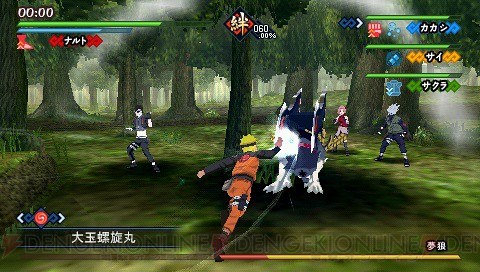The image depicts a retro-style video game screenshot characterized by an Asian language interface, which cannot be deciphered by the viewer. The game's graphical design uses a palette of black, white, red, blue, and green. At the bottom of the screen, there appears to be character or round information displayed in black and white text. The right side displays a 00:00 countdown timer that has expired, accompanied by a green progress bar and a blue progress bar, both three-quarters full. Beneath these bars, red text provides additional, unspecified information. 

On the left side, more system-related text is present, possibly giving stats or instructions. The central area of the screen shows in-game action, where the main character, adorned in orange attire, is engaged in combat with a monstrous opponent. The backdrop for this battle scene is a lush forest, which adds an adventurous atmosphere to the setting.